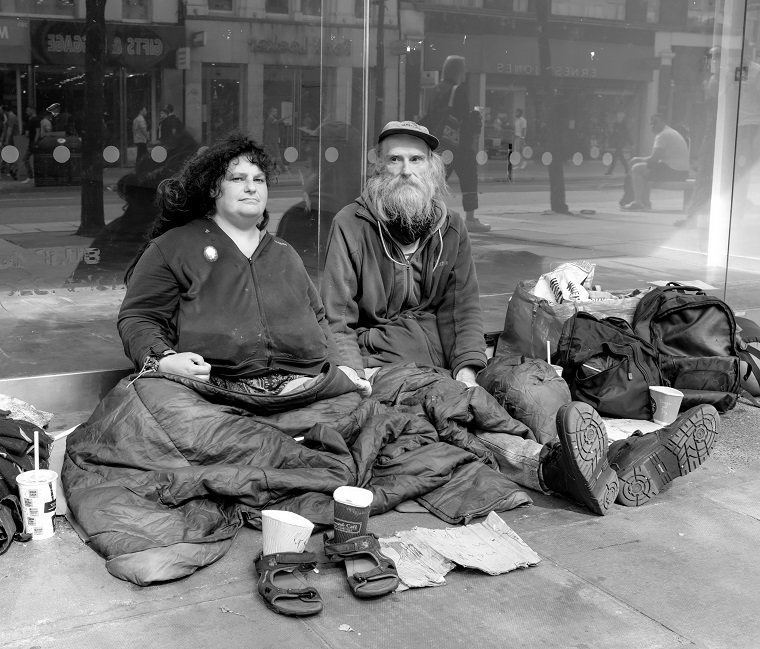A black and white photograph captures a poignant scene of apparent homelessness featuring an older bearded man with gray hair, a mustache, and a baseball cap, sitting alongside a younger, heavyset woman with dark hair. They are seated on a sidewalk in front of a business establishment with large glass windows that reflect pedestrians, trees, and additional storefronts from the street behind them, showcasing a downtown area during late afternoon. Both are dressed in zip-down sweatshirts with nylon jackets draped over their knees. In front of them lie a pair of sandals, several cups, and an unreadable cardboard sign indicative of panhandling. Various bags, including black backpacks, flank them on either side, along with some scattered trash. Their somber expressions and the items surrounding them, such as the shoes placed on the ground, convey their dire situation, hinting at the challenges they face living on the streets.